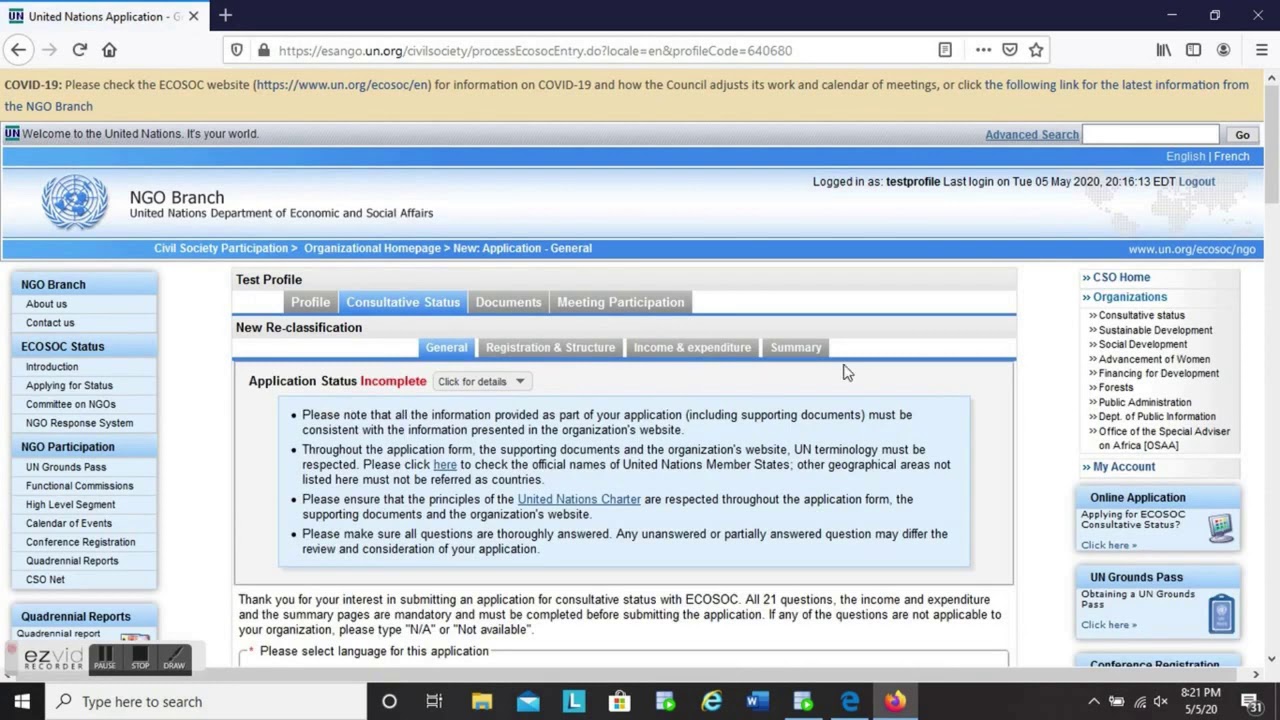The image showcases the application interface for the United Nations Charter on the ESANGO platform, managed by the United Nations Department of Economic and Social Affairs. A COVID-19 warning banner occupies the top of the page against a beige background, providing a link (in blue) to the ECOSOC website for updates on how the pandemic has impacted the council's work and meeting schedules. Additionally, a navigation link to the latest information from the NGO branch is available.

Below this alert, the website URL esango.un.org is displayed, confirming the platform as a part of the United Nations Department of Economic and Social Affairs. The page welcomes users with the message "Welcome to the United Nations, It's Your World", and indicates that the viewer is logged in as a test profile on Tuesday, May 5th, 2020. A logo with a blue background featuring a lighter blue color scheme represents civil society participation.

On the left-hand side of the interface, there are navigation options for various sections, including the NGO branch, ECOSOC status, and NGO participation. The right-hand side lists the viewer's associated organizations. The central segment of the page prominently shows that the application status is labeled "Incomplete" in red letters.

Additionally, the interface extends gratitude to the user for their interest in completing the application and provides further instructions on how to proceed. At the bottom of the page, users are prompted to select the language they wish to use to complete the application. The overall layout emphasizes user interaction and progress tracking for a streamlined application process.